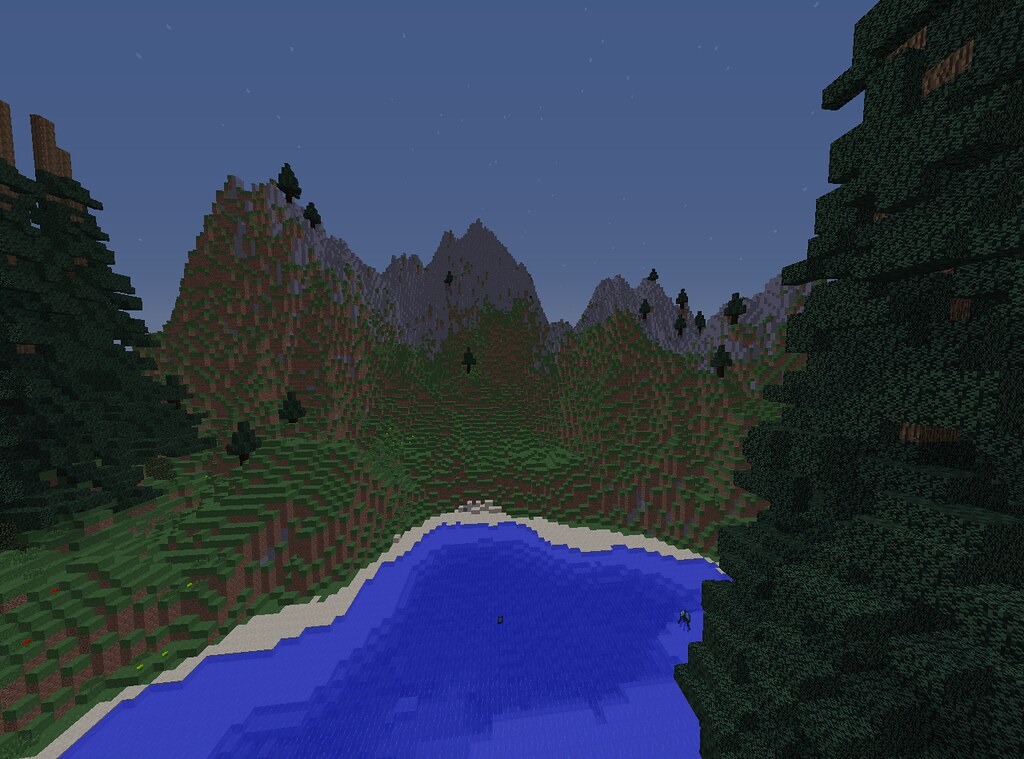In this captivating Minecraft screenshot, we are presented with a sprawling, lush forest teeming with vibrant greenery. The landscape is dotted with undulating hills and majestic mountains, while a serene lake with strikingly blue water occupies the foreground. The water, especially around the edges, appears to be foaming gently, adding a touch of realism to the blocky environment. To the right, close to the camera, stands a tall structure or possibly an imposing tree, contributing a sense of scale to the scene. While there might be aquatic life within the lake, the details remain indistinct. The scene is set during twilight, as the sun has already dipped below the horizon, casting a dim, evening light across the terrain. The entire view exudes the unmistakable charm of Minecraft's pixelated artistry, with its meticulously crafted blocks coming together to form a richly detailed and immersive world.